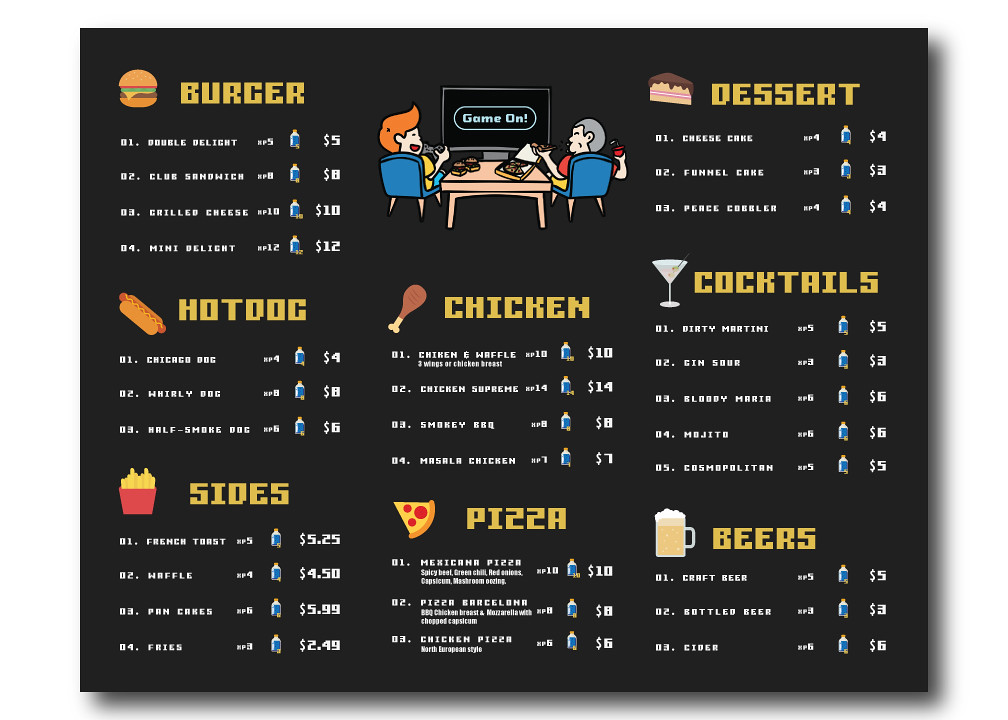This image depicts a food menu likely from a gaming-themed eatery or restaurant. The top of the menu prominently features the phrase "Game On," suggesting that it caters to a gaming crowd or that it's a place to enjoy meals while engaging in gaming activities. The menu includes a variety of food items such as different kinds of burgers, hot dogs, and pizza. There are also sides, desserts, and a selection of beverages including beer and cocktails. The prices are quite reasonable, with burgers starting at $5 and going up to $12, beers priced around $5, and pizzas available for $10. The design of the menu is fairly simplistic with white lettering on a black background, giving it a modern and sleek appearance. Overall, the menu implies an affordable, laid-back spot where people might gather for game nights or casual outings, possibly even bringing their computers or gaming consoles along.